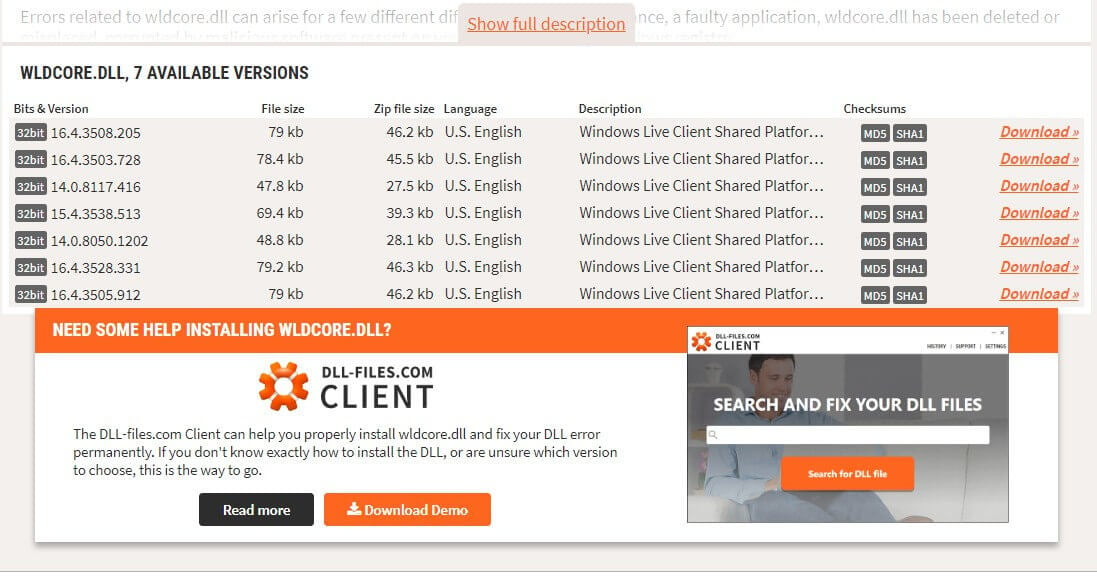**Caption:**

The image showcases a webpage from "wildcore.dll", which provides various versions of the DLL file for download. At the top of the page, there's an orange, underlined link labeled "Show Full Description". Behind this, a partially obscured text mentions that "errors related to Wild Core can arise" due to several reasons, such as a faulty application or the deletion of Wild Core.

The page lists seven available versions of the wildcore.dll file. The table includes columns for "Bits and Version", "File Size", "Zip File Size", and "Language", with all entries indicated in English. Each version is described as the "Windows Live Client Shared Platform". Additional information provided includes check sums like MD5 and SHA-1.

On the right side, there is an orange "Download" button for each version. The site also offers assistance for installing wildcore.dll, suggesting that users can search for and fix DLL files through the site's search bar, highlighted in orange within a client box on the right. This section emphasizes that the DLL-Files.com Client can guide the installation process for those unsure about the correct version or installation method, with further options to "Read More" in a black box or "Download Demo" in an orange box on the left and right sides, respectively.